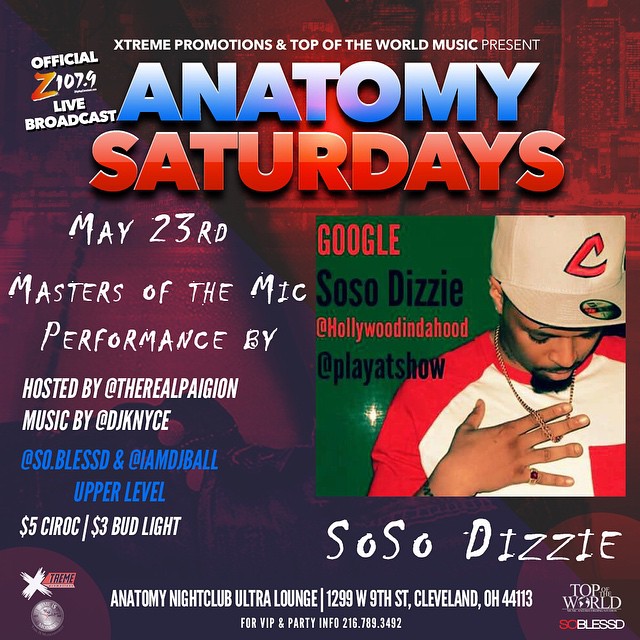Get ready for an electrifying night! Join us for Anatomy Saturdays on May 23rd at Anatomy Nightclub Ultra Lounge (1299 West 9th Street, Cleveland, Ohio, 44113). Witness the Masters of the Mic Performance, hosted by Sosa Dizzy, with a live broadcast by Official Z 107.9. The event is a vibrant mix of red, purple, green, and white, featuring a striking image of a black man wearing a white baseball cap with an orange 'C,' a red and white jersey, and a goatee, looking down with his hand on his chest. Enjoy $5 Ciroc and $3 Bud Light all night. For VIP and party info, call 215-789-3492. Don't miss out on this Top of the World Music and Extreme Productions event!